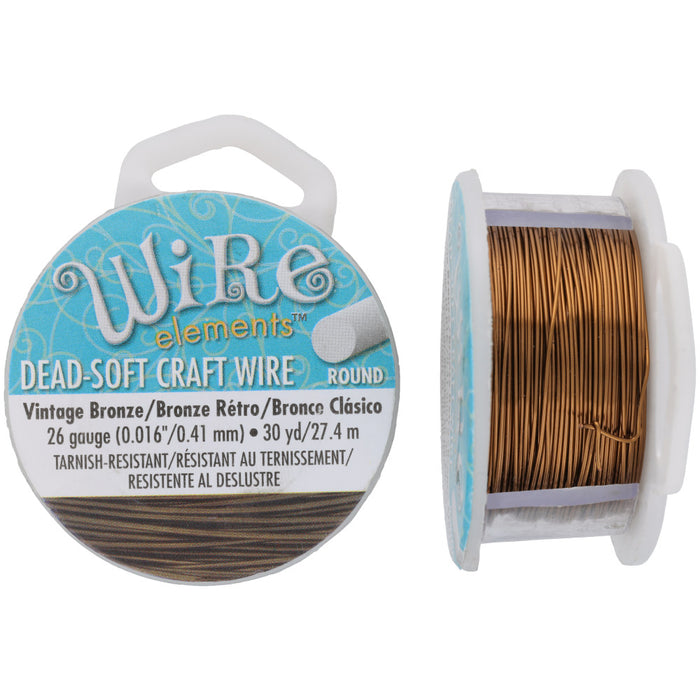The image features a spool of craft wire on a plain white background with no visible borders, presented in two separate pictures. The left picture displays the front of the spool, highlighting its label. The top of the label has a blue background featuring a white spiral design. In white print, it reads "WIRE," followed by "elements" in gold lettering. Below, it specifies "Dead Soft Craft Wire Round" in white print. A white banner beneath this text includes black print detailing the wire type: "Vintage Bronze / Bronze Retro / Bronze Classico, 26 gauge (0.016 inches / 0.41 millimeters), 30 yards / 27.4 meters, Tarnish Resistant / Resistente Deslustre." Underneath this banner, there is an illustration of the wire. The picture on the right shows the side view of the spool, revealing the thin bronze filaments coiled neatly around it. The label is also equipped with a tab at the top featuring an open spot for hanging the spool on a hook.